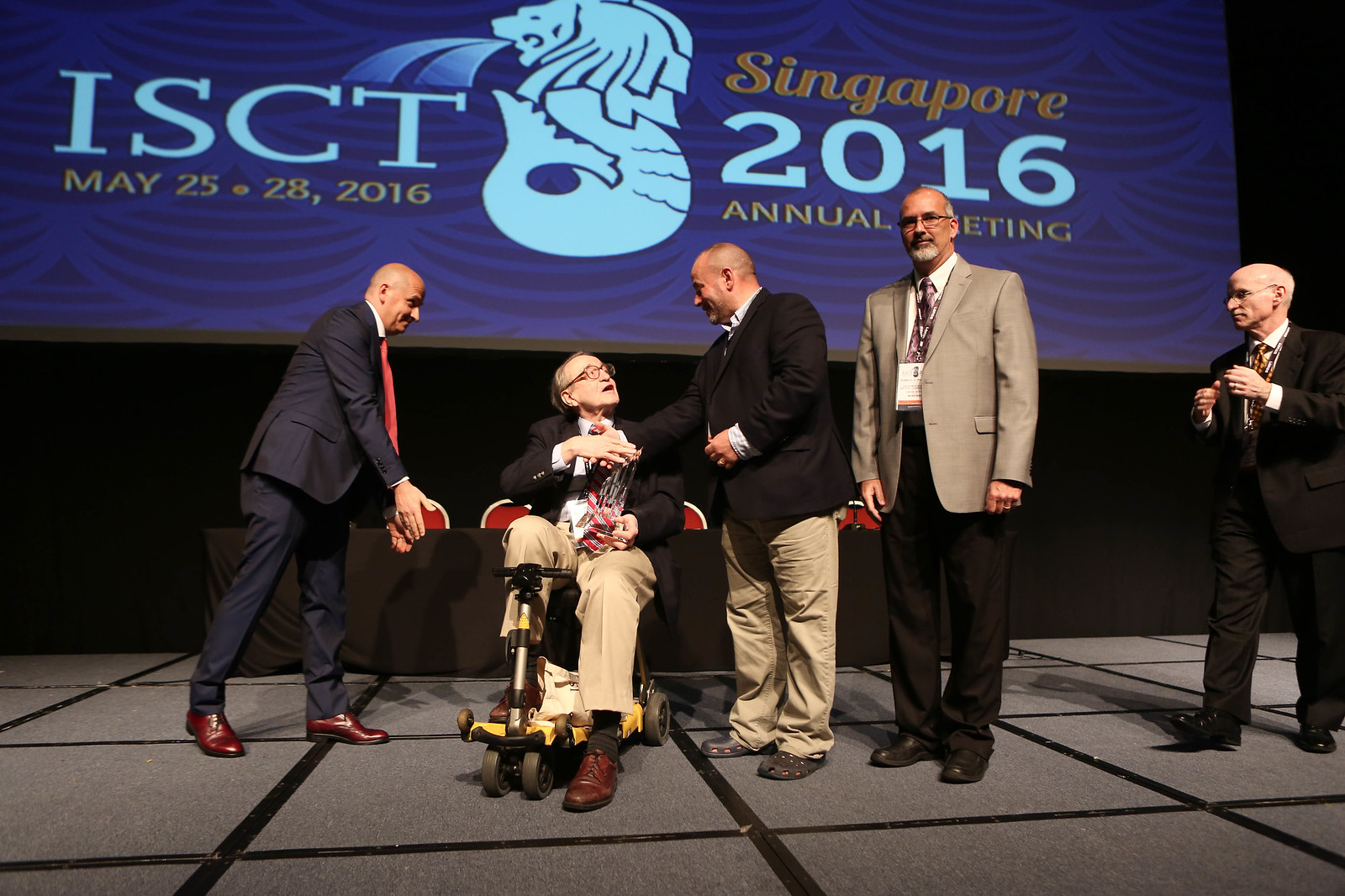In this color landscape photograph, five mature men in business attire stand on a grey stage, set against the backdrop of a blue banner that reads "ISCT Singapore 2016 Annual Meeting," with the dates "May 25-28, 2016" displayed beneath. The central figure is an elderly man seated on a yellow motorized scooter, which has four wheels and handlebars. He is dressed in a dark blazer, shirt and tie, beige pants, and dark brown shoes, with an artificial leg on his right from the knee down, and wears glasses. He extends his hand to shake with a man standing to his left, who is wearing a dark jacket, dress shirt, and beige pants. Another man in a dark business suit with a red tie and white shirt is approaching from the left. To the right of the central figure, a man in a beige blazer, shirt, and tie stands looking ahead, possibly toward the camera. Lastly, another man on the far right is walking towards the group, facing left. All men wear suits, ties, and pass holders around their necks, suggesting they are convention attendees possibly engaged in a congratulatory or formal exchange.